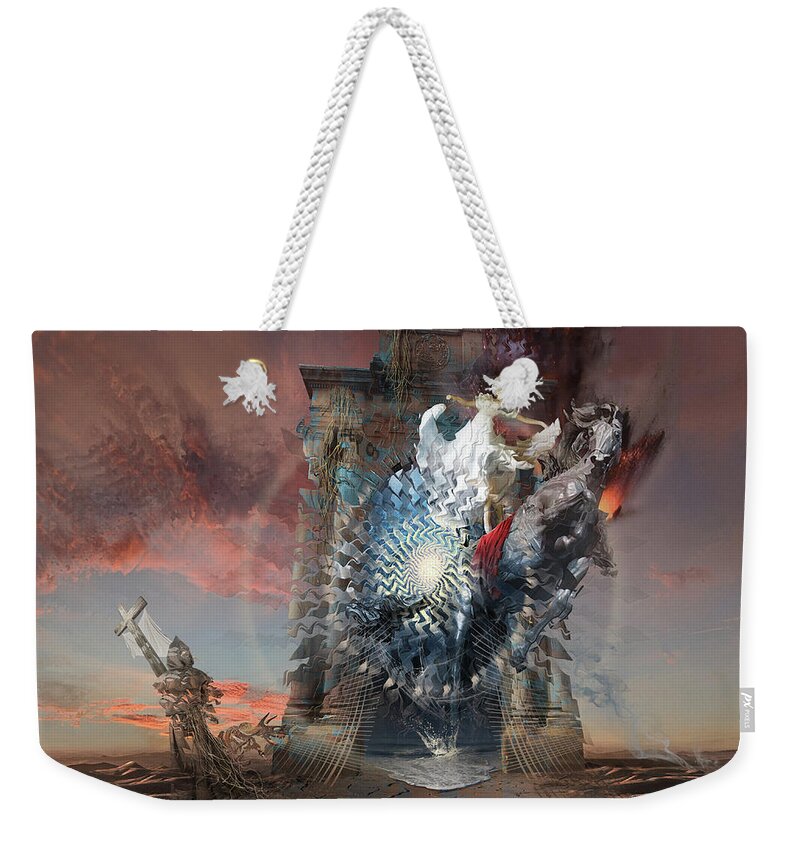This color photograph showcases a tote bag against a solid white backdrop, highlighting its role as a marketplace item. The tote bag, shaped like a purse, features grommets threaded with braided white rope handles, knotted to form simple tassels. The intricate, hand-painted or digitally reproduced artwork on the bag displays a surreal, fantasy-inspired scene. Central to the illustration is a structure evocative of the ancient Arc de Triomphe, appearing to undergo a fantastical explosion. From this arch radiate abstract waves, and emerging from the midst of this chaos is an ill-defined gray horse, almost seeming to be part of the explosion. Additionally, an enigmatic white shape that might resemble an unformed bird is interwoven into the composition.

On the bottom left, a semi-transparent figure, resembling a knight or crusader adorned with a pointed hood, gazes up at the tumultuous spectacle. This knightly figure, which is dissolving, is set against a large Christian cross. To further embellish the surreal ambience, the painting's background portrays a vibrant sky, mixing watery watercolor blues with pinks, purples, and light-colored clouds, culminating in a strikingly imaginative and science fiction-esque visual narrative. Low mountains are faintly visible in the distant background, adding depth to this fantastical landscape.